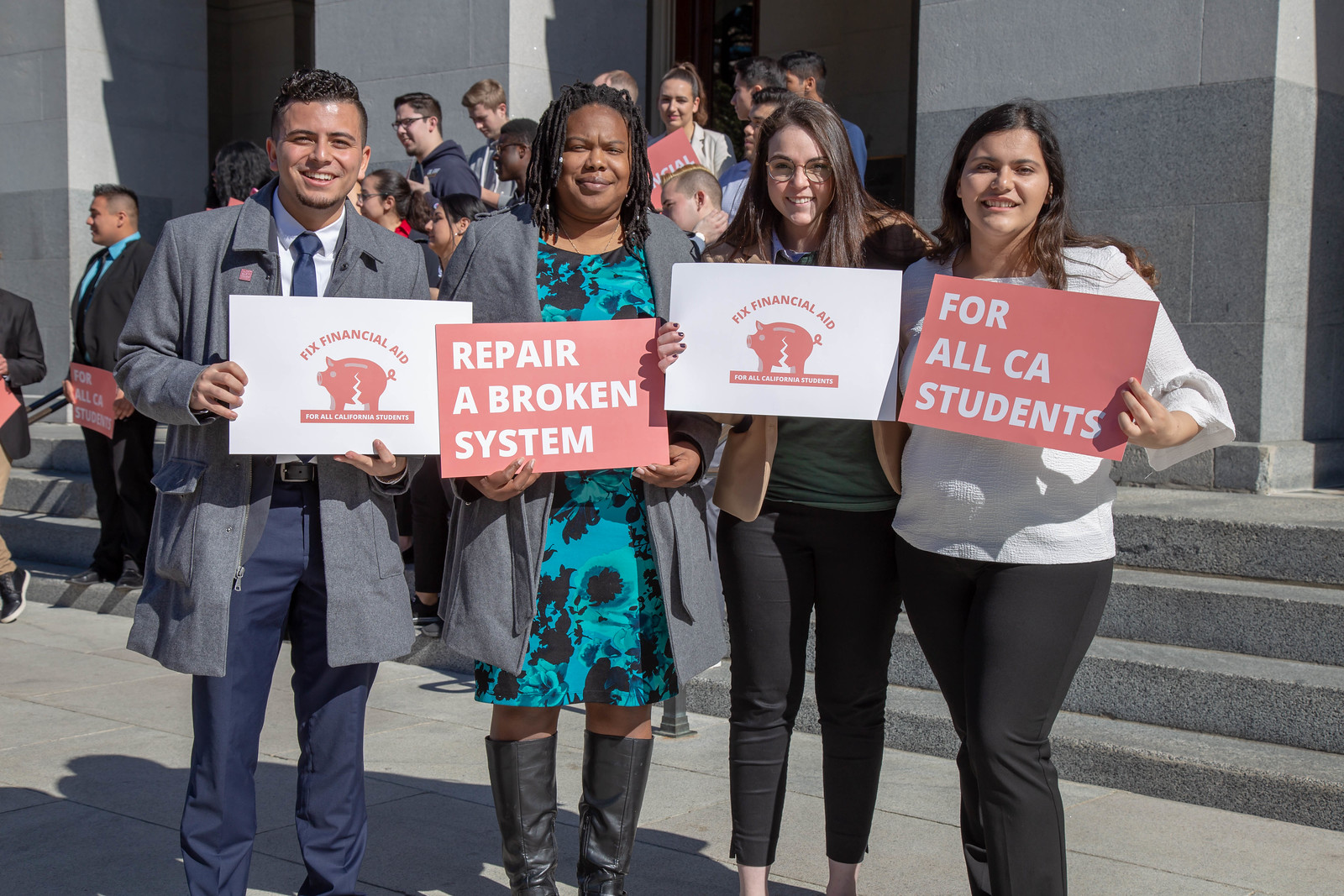The photograph captures a vibrant protest scene advocating for the reform of California's financial aid system. At the forefront, four individuals stand resolutely on the steps of a light gray stone building. They each hold small yet impactful signs. The man on the left, dressed in a blue shirt and tie, a Latino, holds a sign displaying a cracked red piggy bank with the words "Fix Financial Aid". Next to him, an African American woman holds a red sign with bold white text that reads "Repair a Broken System". The third protester, a woman, holds a sign identical to the first man's, reiterating the call to "Fix Financial Aid". The final demonstrator on the far right, a woman, hoists a red sign declaring, "For All CA Students". Behind these four leaders, a diverse crowd of about 15-30 people from various ethnicities, nationalities, and religions can be seen. They are united in their demand for a fair and functional financial aid system for all California students.